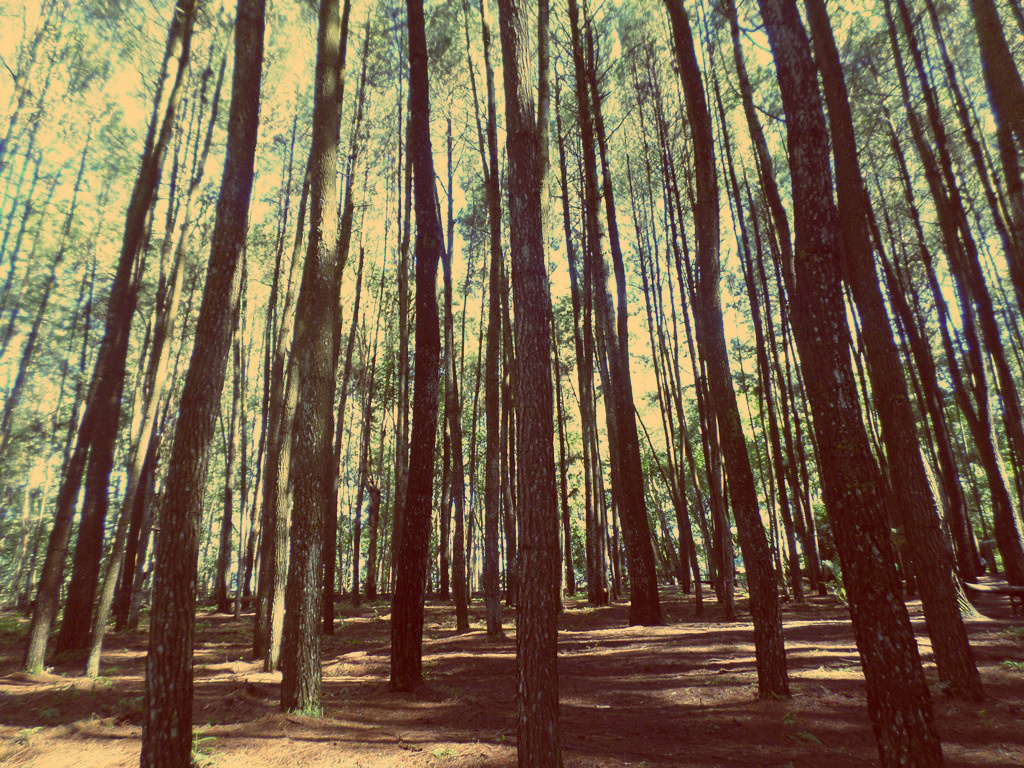This realistic color photograph captures an outdoor daytime scene inside a dense forest. Taken from a kneeling viewpoint, the image looks upwards through a thicket of very tall, slender trees, all uniform in size with thin trunks. The canopy of leaves is high above, allowing an orange-tinged sky to peek through. Sunlight filters down, creating patches of white and gold on the predominantly brown soil of the forest floor. The ground is a mix of dirt, with sparse brown leaves and some weeds scattered about. The trees are densely packed, leaving little room for movement without caution. The predominant colors in the image are green and brown, with hints of white and gold from the sunlight. Though some might describe it as having a sepia-like filter, the natural colors still shine through, giving it a vibrant yet earthy feel.